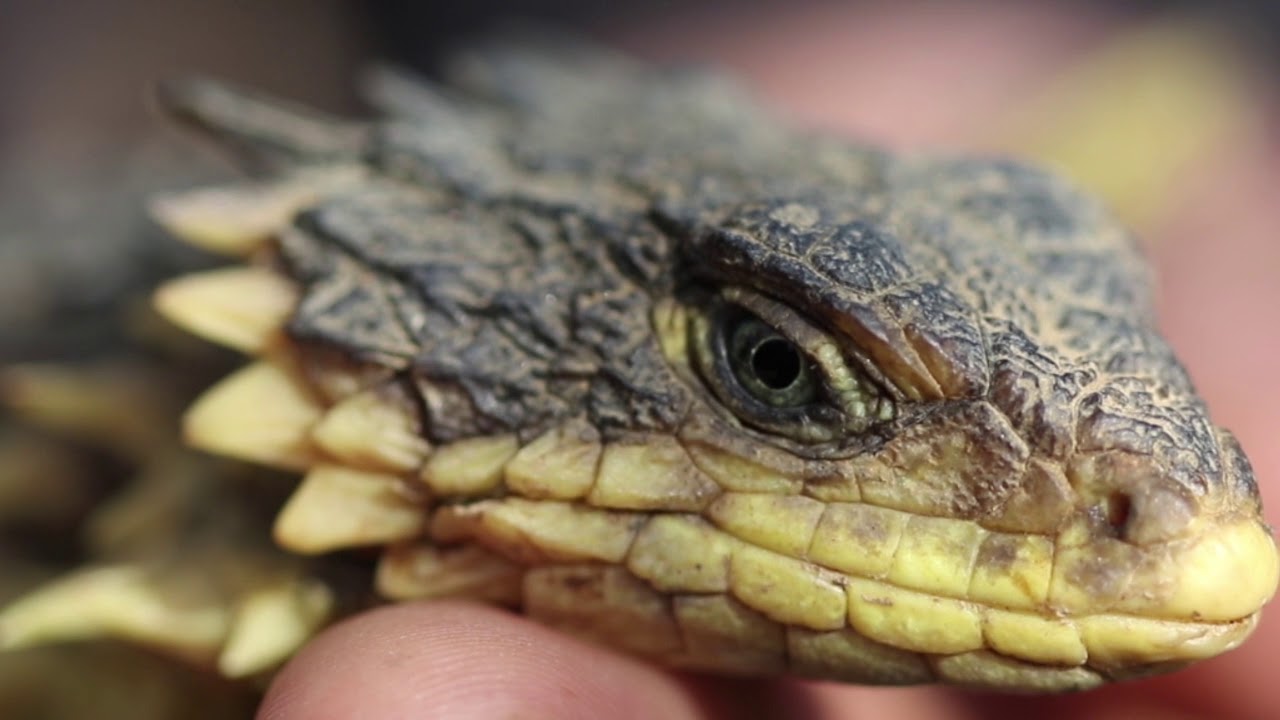The photograph showcases a close-up of a lizard's head with a sharply blurred background. The head, prominently featured, is primarily dark gray to black with a hint of green. The top of the head is black, transitioning to a yellowish hue along the jawline and the mouth. The lizard's eyes are round, predominantly black with a gold ring encircling the central pupil. Behind the head, a ruffled segment with ragged scales stands out, displaying a cream color. Every wrinkle and scale of the lizard is visible, enhancing the textured detail of its skin. The head is somewhat flat and ends in a pointed snout. The background, although largely indistinct, contains subtle hues of gray, green, yellow, and purple, adding a faint but colorful context to the striking portrait of the lizard, which gazes sideways out of the frame.